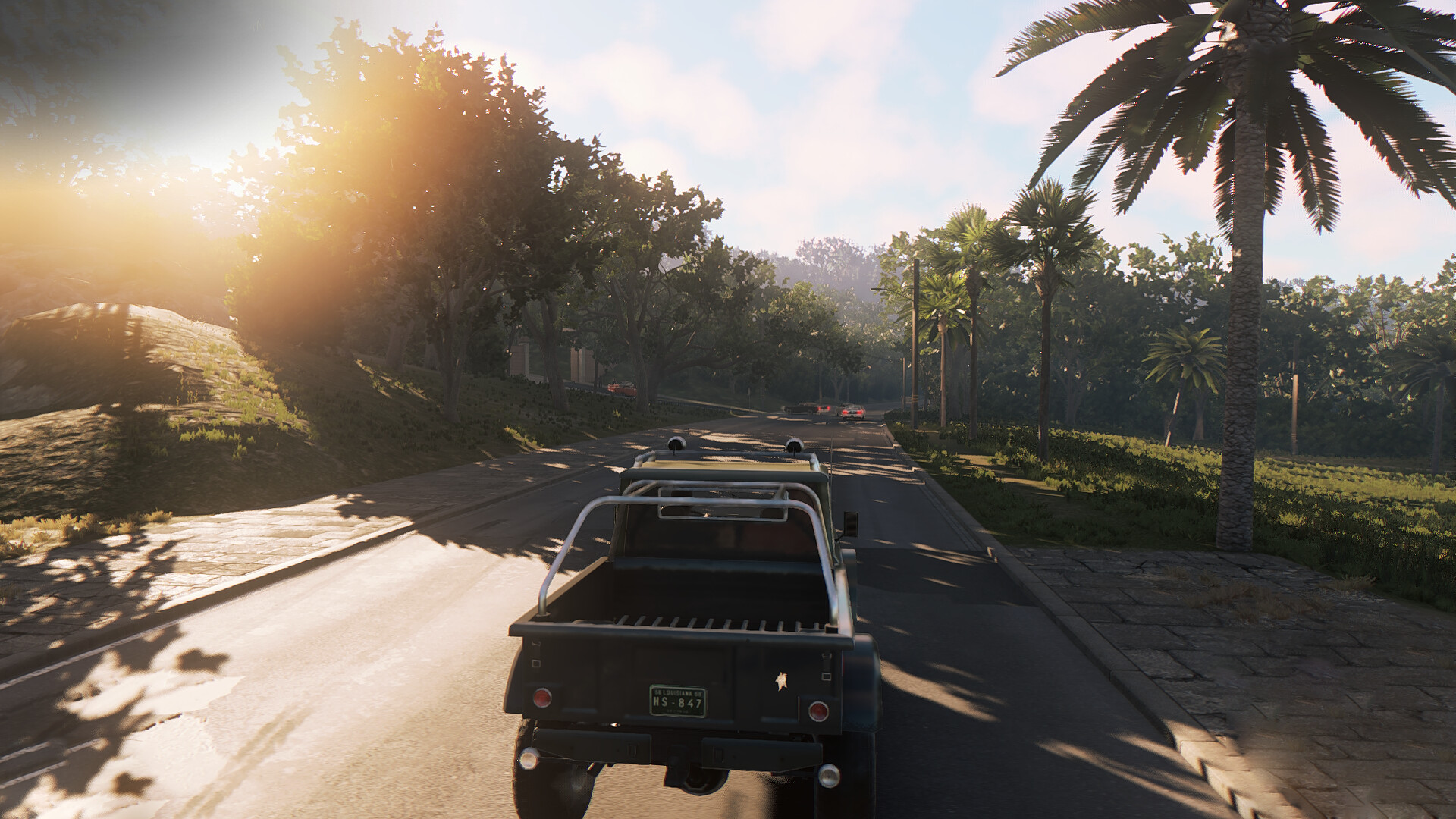A highly-detailed, possibly computer-generated image depicts an old, charcoal gray truck driving down a street. The truck is adorned with a green license plate, marked with partially legible characters that read either "HS 847" or "NS 847"; the state is indistinguishable. The high-resolution scene features a road flanked by lush palm trees on the right and a landscaped area with paver stones on the left. A gentle hill rises in the background, dotted with what appear to be deciduous trees. The sky is a vibrant blue, filled with fluffy white clouds, and a peculiar sunburst effect illuminates the top left corner, adding an almost artificial glow to the scene.